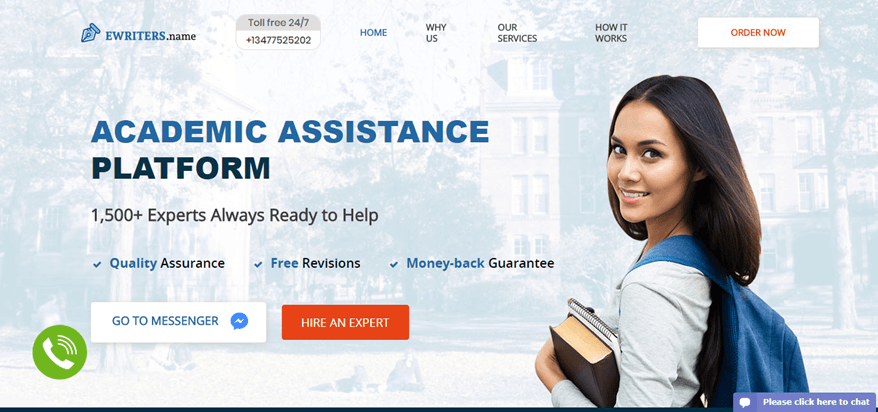This landscape-oriented advertisement, much longer than it is tall, evidently promotes the eWriters.name website or program. The background features a grayed-out image of a picturesque college campus with tall buildings, brick houses, giant trees, and winding pathways. At the top, the logo displays a pen tip icon accompanied by the text "eWriters.name" in blue. Just beneath the logo, a gray and white box provides a toll-free 24-7 phone number.

Below this section, a navigation menu features links such as "Home" (highlighted in blue), "Why Us," "Our Services," and "How It Works" in black. Adjacent to these links is a prominent white box with orange text urging viewers to "Order Now."

The main body of the advertisement presents the phrase "Academic Assistance" in blue, followed by "Platform" in a darker blue. It boasts "1500+ experts always ready to help" and assures potential users with promises of "Quality Assurance," "Free Revisions," and a "Money Back Guarantee."

Towards the bottom, a green circle with a white phone icon symbolizes connectivity, accompanied by a white box with blue text reading "Go to Messenger" and a chat bubble. An adjacent orange box with white text invites users to "Hire an Expert."

To the right of these elements is an image of a smiling young lady. She has a darker complexion, long brown or black hair, and is dressed in a white long-sleeved shirt. She carries a backpack and holds two books, looking directly at the camera.